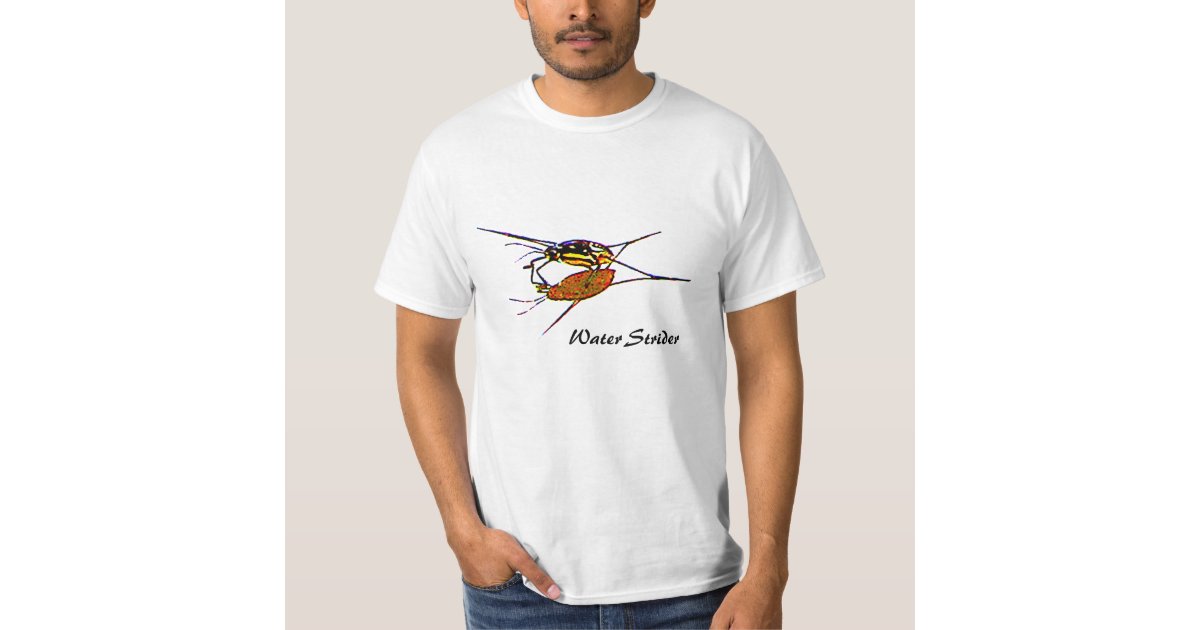The image is a professionally taken, full-color, square photograph, likely from a website advertising the t-shirt. It features a tan, brown-skinned man with a very thin beard and mustache, standing indoors against a grayish-white background. The man is partially cropped, visible from just below his eyes to his hips, dressed in blue denim jeans with one hand tucked into his pocket. He wears a bright white, short-sleeved, ring-neck t-shirt with black text that reads "Water Strider" beneath a colorful drawing of a black, yellow, white, and red insect atop another bug, which appears to be brown, black, orange, and green in color. The artistic design on the t-shirt creates ambiguity, possibly resembling a shadow or another object.